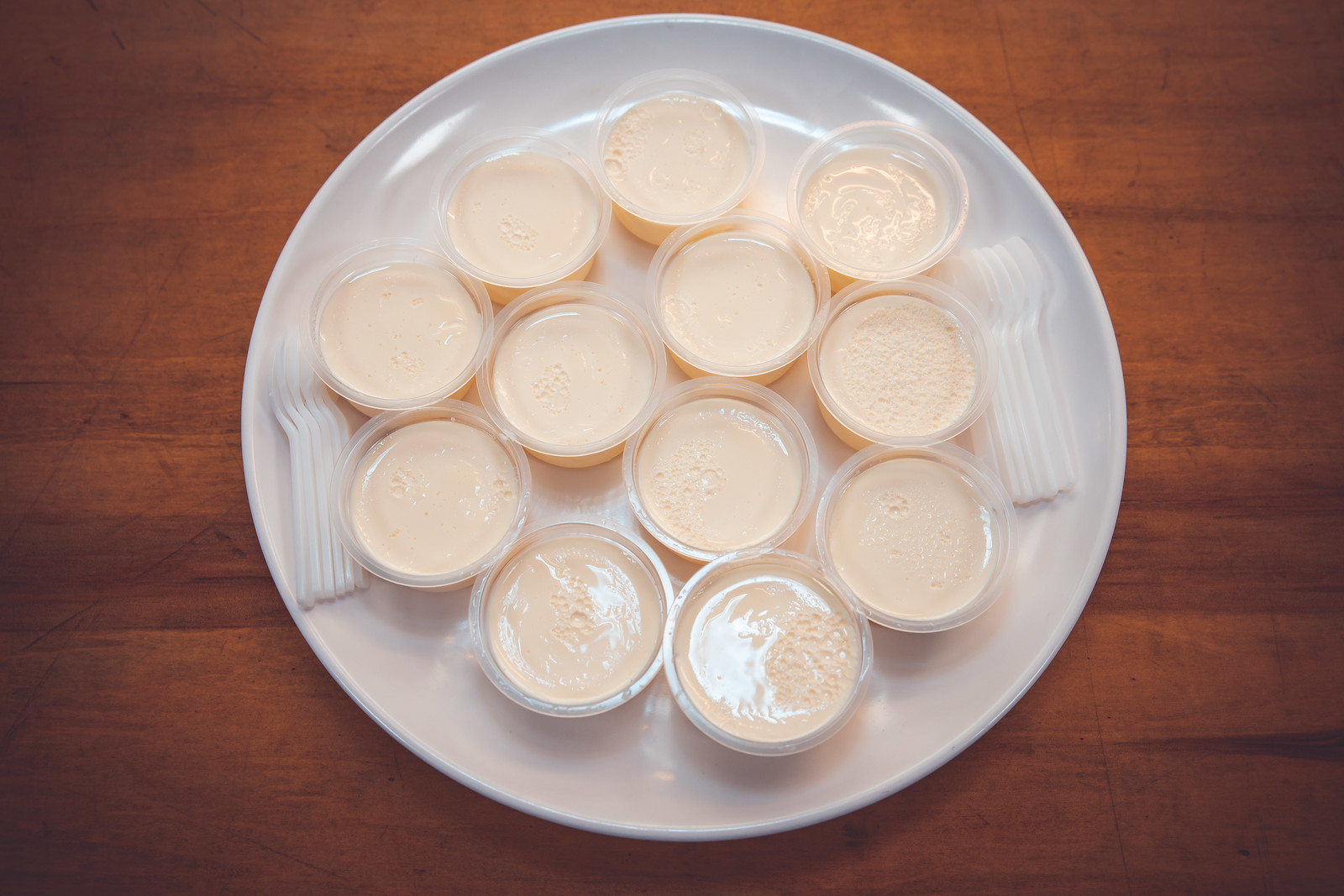The image displays a white, round plate with a subtle lip, centered on a mid-tone brown wooden tabletop that shows noticeable grain patterns, scratches, and imperfections. Arranged neatly on the plate are twelve small white plastic condiment cups, each containing a cream-colored substance, likely pudding, custard, or a similar gel-like dessert. The surface of the contents has small air bubbles and appears evenly settled. Flanking the cups on both the left and right sides of the plate are rows of four miniature white plastic spoons, positioned at approximately the three and nine o'clock positions. The spoons are aligned with their bowls facing the central row of cups, creating a symmetrical and orderly presentation.